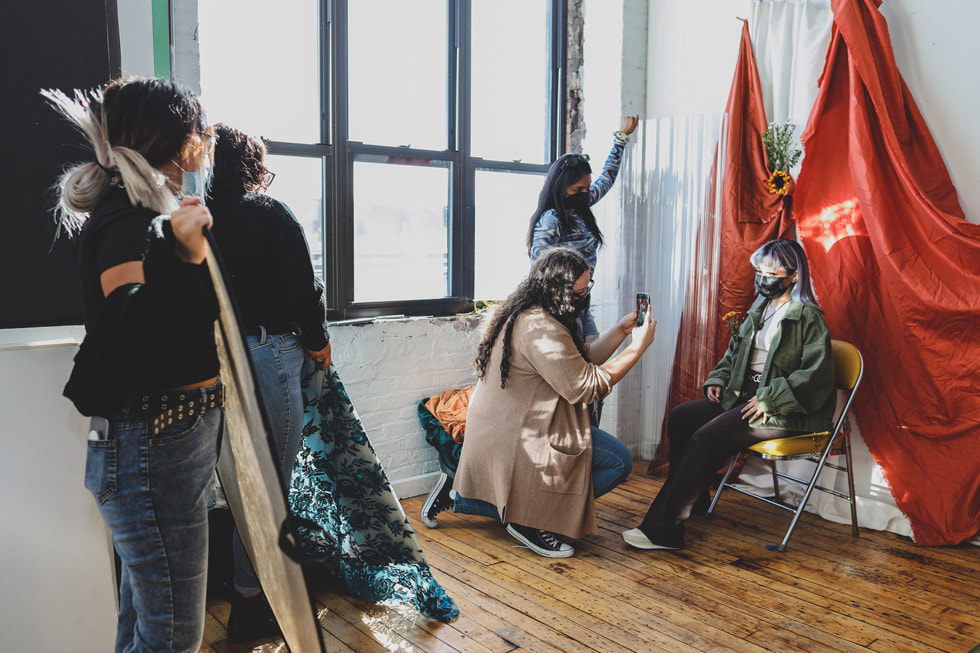This detailed photograph depicts a behind-the-scenes moment of a photo session in an artsy, warehouse-style room with a yellow wood floor and white-painted brick walls. Dominating the background are three large, vertical, rectangular windows with black borders, bathed in intense natural light. Central to the image is a young woman with streaked white and black hair, sitting in a small folding chair with a yellow padded seat and backrest. She wears a green army-style jacket, dark-colored pants, and running shoes. 

All participants in the image are wearing N95-style masks, indicating a COVID-era shoot. The woman seated in the chair is the focal point, surrounded by a dynamic red drapery cinched in the middle, resembling an M shape, with a yellow scrunchie supporting fur-like branches at its center.

To her immediate front, a woman with long curly hair, bespectacled, and wearing a beige coat, blue jeans, and black-and-white Converse sneakers kneels, holding a smartphone to capture the shot. Another woman, standing just behind her to the left, wears a blue psychedelic-patterned shirt, has black hair with glasses perched on top, and is holding a large piece of see-through, corrugated plastic.

Further left in the frame, one woman holds a floral-patterned green fabric, wearing jeans and a dark long-sleeved shirt, while the furthest left figure, dressed in a black shirt and blue jeans, holds a light reflector. The bright sunlight pouring through the blown-out windows sharpens the contrast and illuminates the room, emphasizing the creative energy and meticulous preparation of the scene.